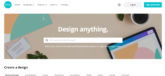A screenshot of a website with an interface resembling a graphic design platform, possibly similar to Canva or Cricut. The image is slightly blurry, making the main heading difficult to read, but it appears small in size. The central section of the page features a colorful display, including elements that resemble a tablet and various design tools. Above a prominent search bar, the phrase "Design Anything" is clearly visible, and beneath it, a slightly obscured tagline appears to say "Create a Thing." The overall layout and elements suggest a user-friendly design website where users can create custom products or designs.